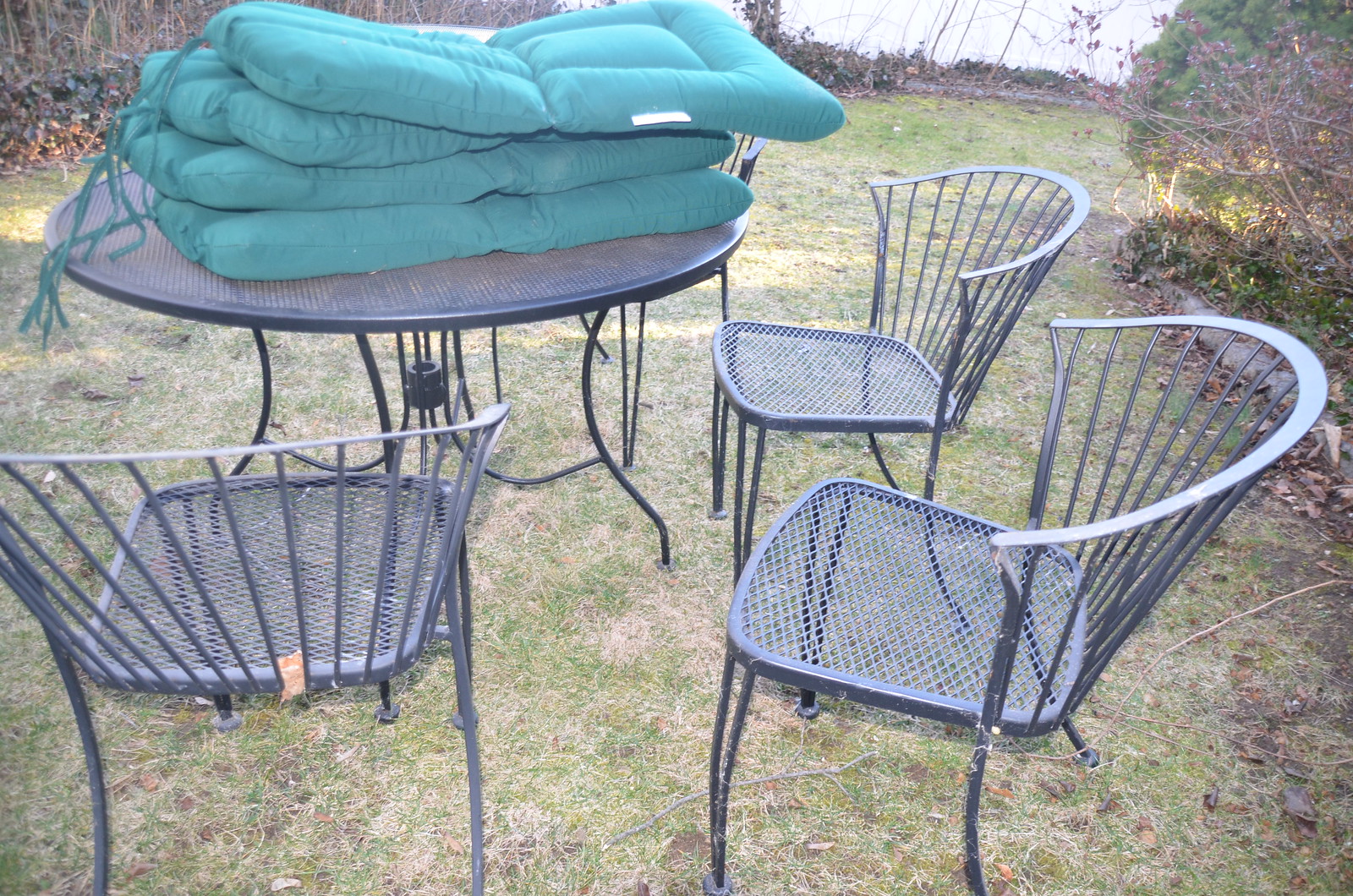The image depicts a horizontal rectangular photograph of a concrete patio area featuring outdoor furniture. There are three gray metal chairs and a matching gray metal table that has a hole in the center for an umbrella, although no umbrella is present. Four aqua-colored seat cushions with ties are stacked on top of the table, presumably to be fastened to the chairs for added comfort, given that the chairs are made of hard metal. The setting appears somewhat barren as the grass visible beyond the patio is sparse and interspersed with patches of dirt. Some landscaping is visible on one side, adding a touch of greenery to the scene.